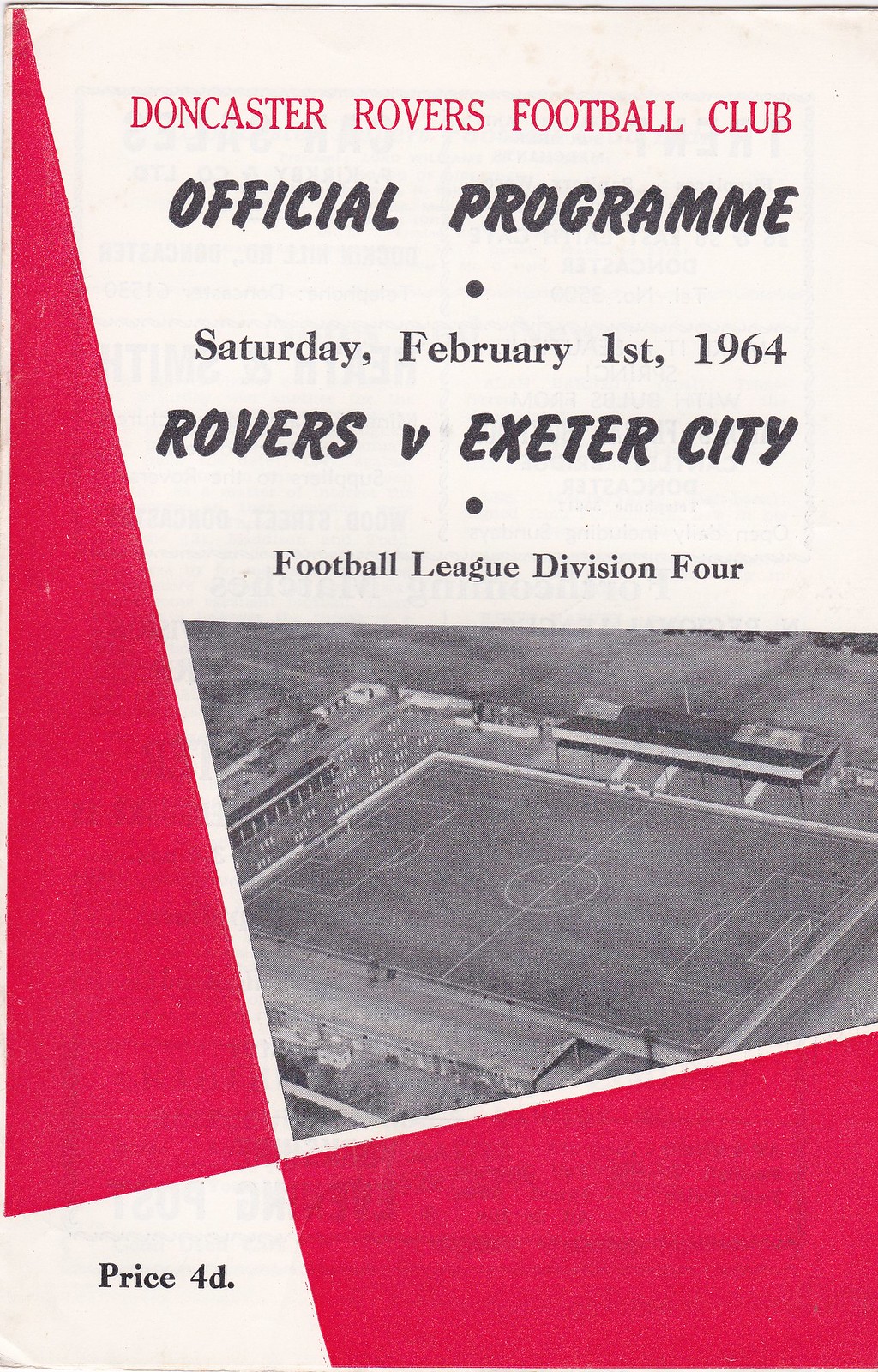The image showcases the front cover of an official program from the Doncaster Rovers Football Club. At the top, the cover reads, "Doncaster Rovers Football Club Official Program, Saturday, February 1st, 1964: Rovers vs. Exeter City, Football League Division 4." Below this text, the price of the program, "Price 4D," is displayed in the bottom left corner. The central focus of the cover is a photograph depicting a football field. The overall color scheme includes shades of purple, tan, black, white, and various grays. The layout is clean and organized, with most of the text positioned at the top, the photograph centrally placed, and the price noted at the bottom left. The style and presentation suggest it is an official matchday program, typically purchased by fans attending the soccer game in person, reflecting the era's design aesthetics.